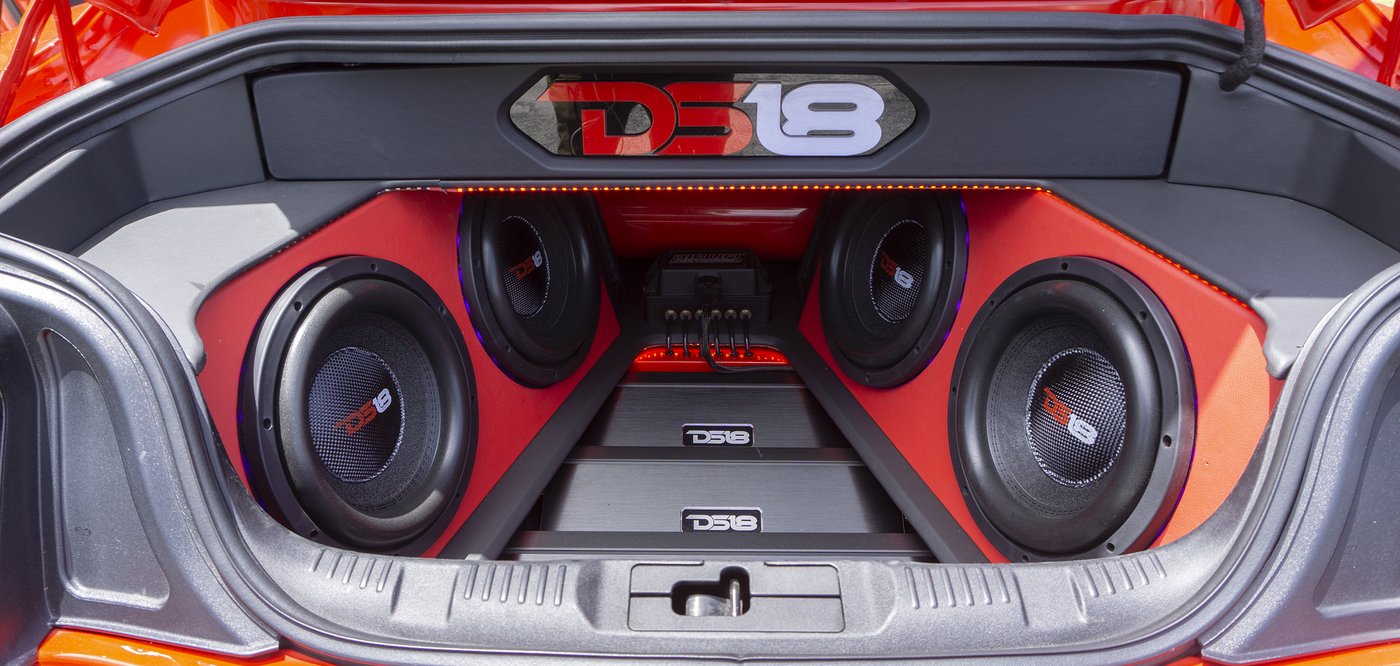This detailed landscape image showcases the trunk of a red car, which has been lifted open to reveal an elaborate and professionally installed DS18 sound system. At the top of the trunk area, the brand name DS18 is prominently displayed, with the letters "DS" in red and the number "18" in an off-white color. The trunk houses four large speakers, with two positioned on the left and two on the right, all featuring black interiors and reddish-orange accents outlining them. Below the speakers, at the very bottom end of the trunk, there are a couple of subwoofers and visible electronics where everything plugs in, including power connectors and possibly even extra battery power. Designed to advertise its high-performance capabilities, this custom setup hints at a powerful sound experience capable of making the vehicle vibrate with impressive audio intensity. The colors in the trunk area are primarily red, black, and gray, enhancing the sound system's bold and stylish appearance.